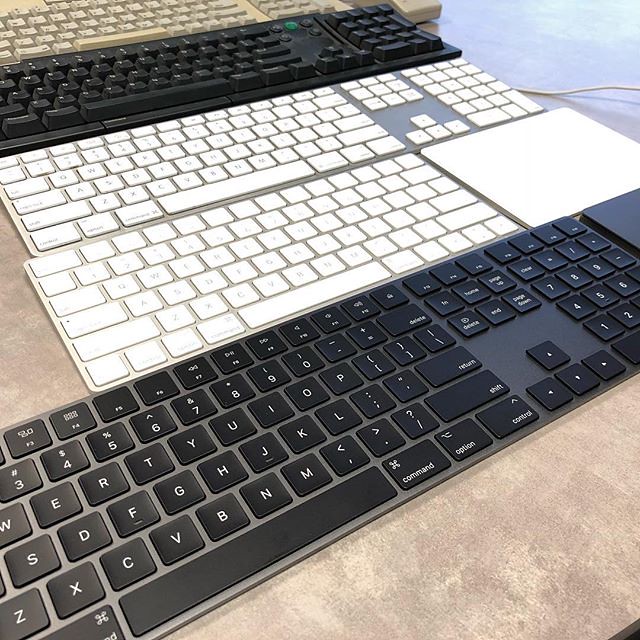The image showcases five keyboards laid out on a laminate countertop with a granite-like appearance. In the foreground, there is a sleek, black keyboard with white letters. Directly behind it is a silver Apple keyboard with white chiclet keys, featuring a blank white section to the right. The next keyboard up is another Apple keyboard, similar in design with chiclet keys but featuring a full number pad. Above this is a black keyboard with a green button, characterized by raised keys suggestive of a mechanical type. The final keyboard in the background is a dingy tan color, appearing old and reminiscent of classic office keyboards. The arrangement creates a visually interesting sequence of black, white, and tan colors on a neutral surface, lending a tactile and organized impression to the photo.